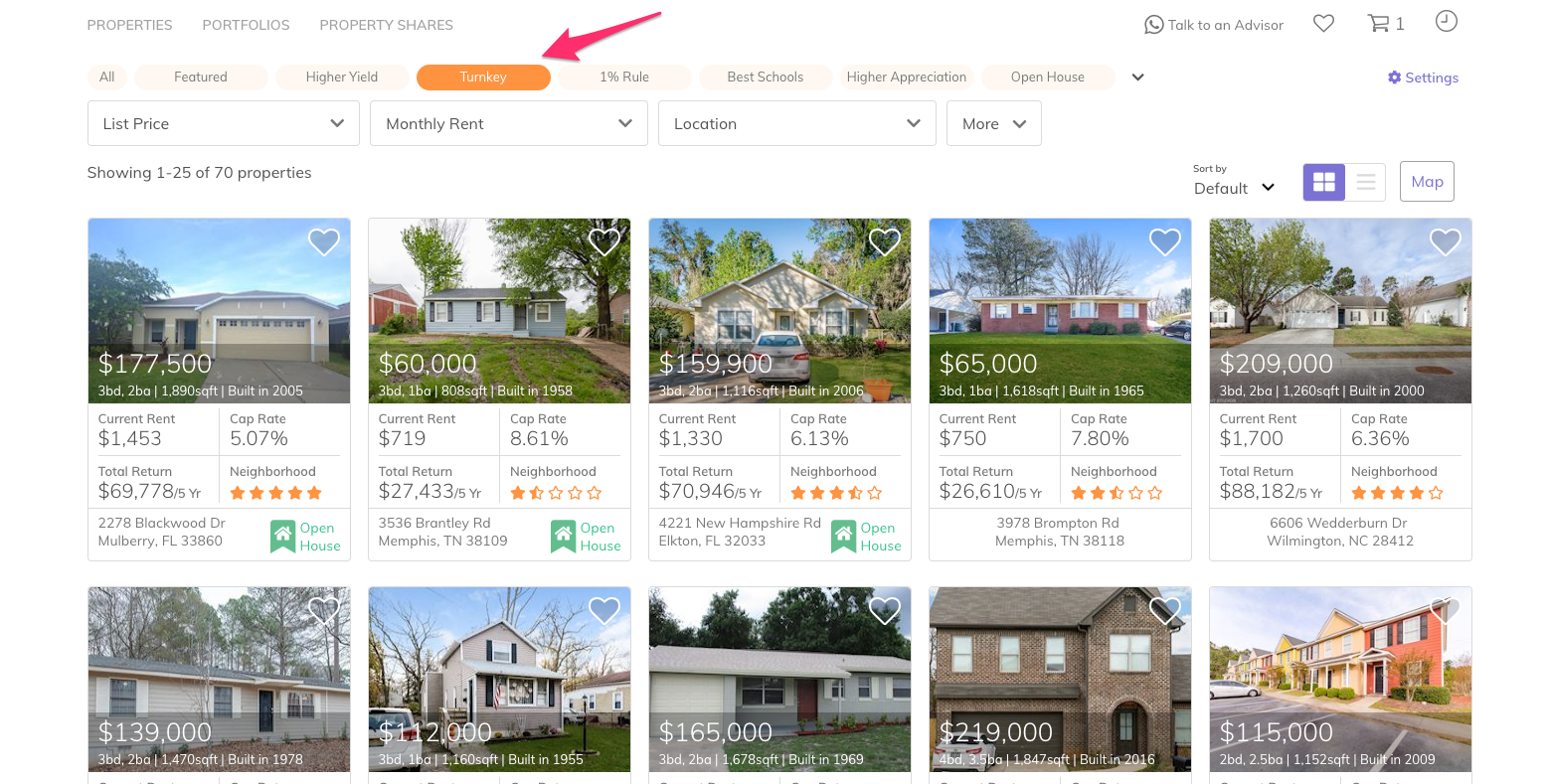The user interface displays three words in gray, uppercase text in the top-left corner, offering three distinct choices. Below these options, there are eight light tan, oval-shaped buttons arranged horizontally. The fourth button from the left is selected, displaying "TURN KEY" in white text. A pink arrow originating from the top-right corner diagonally points towards the "TURN KEY" button. 

In the top-right section, there is an option labeled "Talk to an Advisor" accompanied by a phone icon. Adjacent to this are three additional icons: a gray-outlined heart, a gray shopping cart with a notification indicating one item, and a gray clock. Below this row of icons lies a purple gear icon labeled "Settings."

Beneath the settings icon, the interface houses four drop-down options within gray rectangles. Following these drop-down menus, a section labeled "Properties" showcases several property listings. Each listing features an image with a white-outlined heart icon at the top right. The properties are detailed with their price, current rent, cap rate, total return, and neighborhood rating. The neighborhood rating is highlighted with a five-star system rendered in orange.